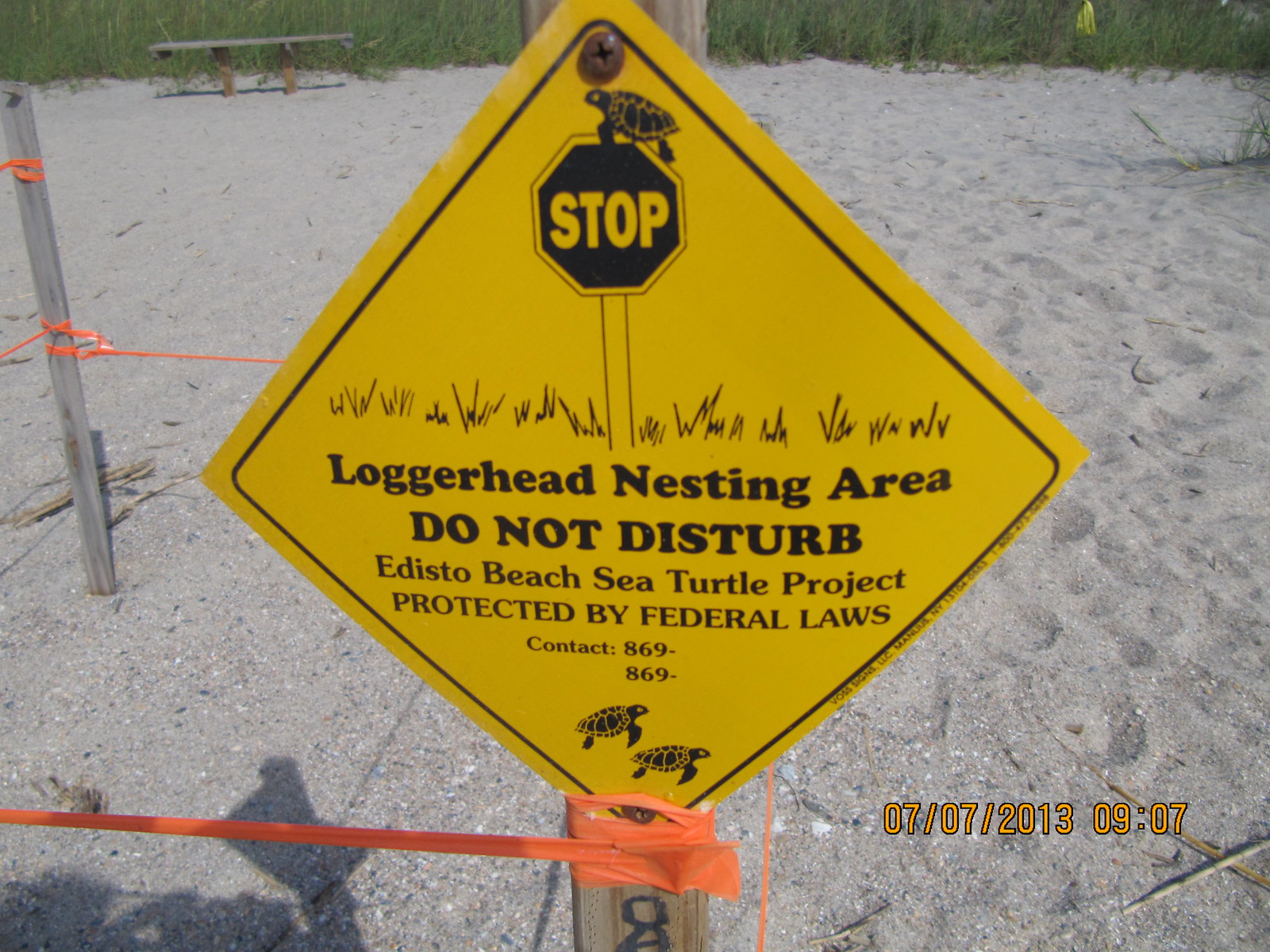The image is a detailed photograph of a yellow, diamond-shaped sign affixed to a wooden pole, situated in a beach area with rough sand in the background. The sign, which has a dark border, prominently displays a black ink illustration of a turtle perched on top of a stop sign, with some grassy elements around it. Below this illustration, the text reads, "Loggerhead nesting area, do not disturb. Edisto Beach Sea Turtle Project, protected by federal laws," followed by an area where contact phone numbers are to be written, currently listed as "contact 869-869." At the bottom of the sign are two more turtle illustrations. The sign is part of a small enclosure made by red plastic bands connecting multiple poles, presumably to prevent people from entering the protected nesting area. In the background, you can see a wooden bench and tall green grass, contributing to the natural beach setting. Additionally, in the bottom right corner of the image, orange text indicates the date and time: "07/07/2013 09:07."